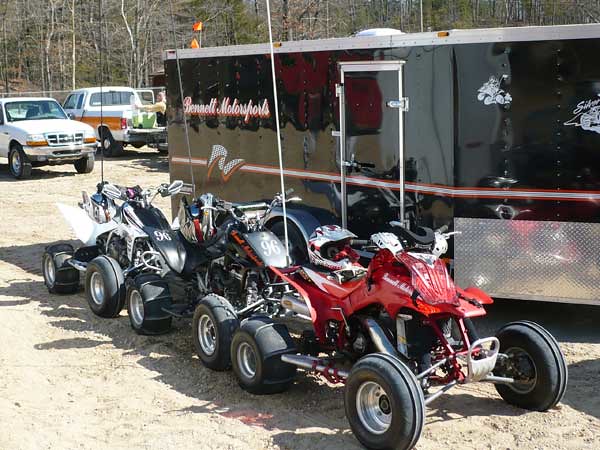Outdoor color photograph in landscape format showcasing a sandy parking area with several ATVs and vehicles. The main focus is on a line of four ATVs sitting on a dirt road. The first ATV is red with a white helmet on its seat, followed by a black ATV with the number 96 beneath the handlebars, another black ATV also with the number 96, and a predominantly white and black ATV at the end. These ATVs are vertically lined up, with two facing one direction and the other two facing the opposite direction. Behind the ATVs is a black trailer with a pink and white pinstripe down the center, aluminum grating at the front, and the words "Bennett Motorsports" in white and orange cursive. Beyond the trailer, there are two white pickup trucks parked, and the background is lined with mostly bare trees, some still bearing green leaves. The ground is light gray, rocky gravel casting shadows from the ATVs, creating a rugged outdoor scene.